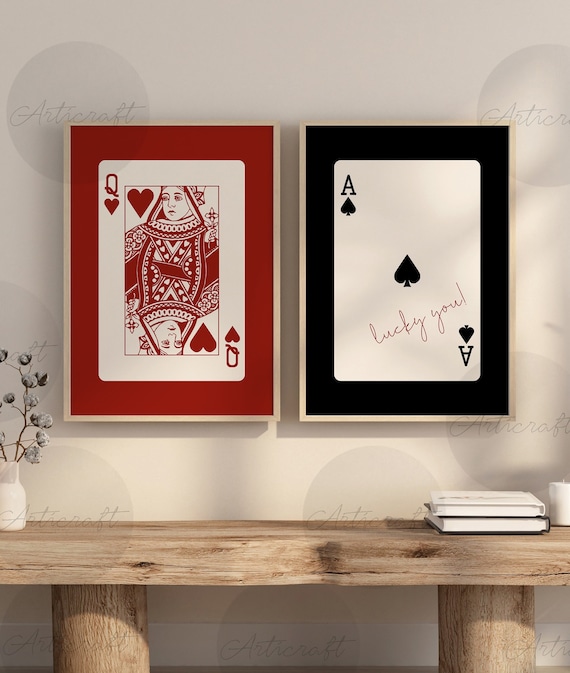The photograph showcases a section of someone's home, focusing on decorative elements against a beige wall. At the center of the image, two large framed pieces of art depict playing cards—a Queen of Hearts on the left with a red background and gold frame, and an Ace of Spades on the right with a black background and gold frame. The Queen of Hearts card shows the traditional dual images, straight up and upside down. The Ace of Spades features the text "Lucky You" in cursive on the bottom right. Below these artworks is a modern, light wood table supported by legs resembling tree trunks. On the table are two books, a white candle, and a white vase containing what appears to be an artificial plant or cotton blooms. The arrangement is minimalist yet striking, accentuated by a watermark for AstroCraft in the corner.